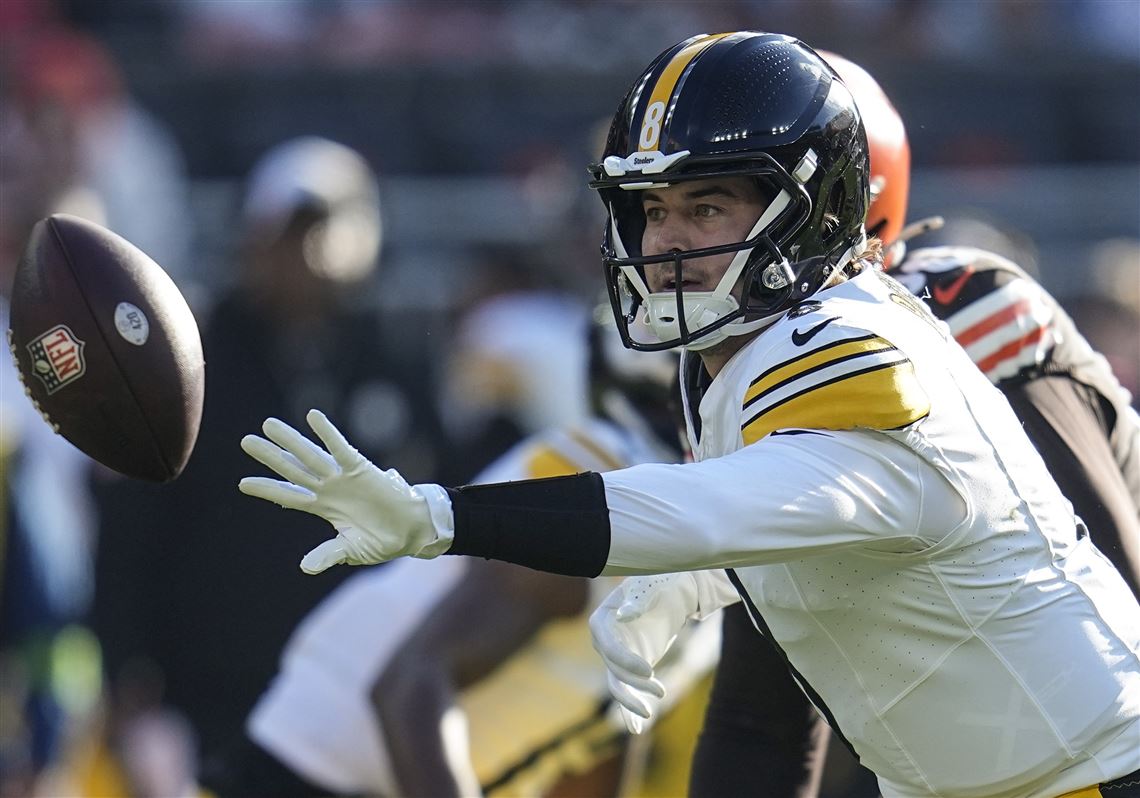An outdoor color photograph captures a dynamic moment in an American football game. The image's primary focus is on a young football player, approximately 20-22 years old, who is leaning into the frame from the right side. His left arm is fully extended, fingers outstretched towards a brown, vertically oriented NFL football that is mid-air on the left side of the image. He wears a blue helmet with a gold stripe and the number 8 emblazoned on it, partially shadowed by the sunlight. His face, though partially obscured by the helmet's guard, reveals brown eyes, white skin, and a hint of a moustache.

The player is dressed in a white jersey featuring a Nike swoosh on the left shoulder and a yellow stripe running along the shoulder pads. White gloves cover his extended left hand, while his bent right arm, marked with a black armband, is visible just below his left elbow. Behind him, another player dressed in black with a red helmet appears, though their face is not visible. The background is a blur of indistinct figures and colors, focusing attention solely on the central action of number 8 reaching for the football.